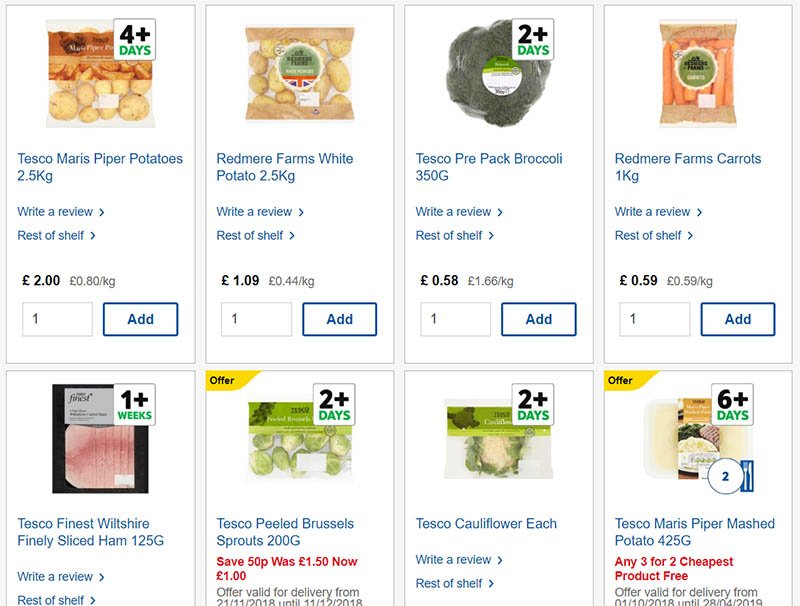Screenshot from a Grocery Website:

The screenshot depicts a portion of a grocery website, displaying eight product listings on a plain white background. Due to the partial capture, the bottom of the image is slightly cut off, and some elements are not fully visible. Each product is displayed within vertical rectangular boxes.

From left to right, the products are categorized as follows:

1. **Tesco Maris Piper Potatoes**:
   - Image: Bag of potatoes
   - Description: Tesco Maris Piper Potatoes with weight mentioned
   - Features: Options for writing a review, viewing the rest of the shelf
   - Price: $2
   - Additional Elements: Quantity box (set to 1), 'Add' button

2. **Red Mirror Farms White Potatoes**:
   - Image: Bag of white potatoes
   - Description: Red Mirror Farms White Potatoes
   - Features: Write a review, rest of the shelf
   - Price: $2
   - Additional Elements: Quantity box, 'Add' button

3. **Tesco Pre-packed Broccoli**:
   - Image: Broccoli head
   - Description: Tesco Pre-packed Broccoli
   - Features: Write a review, rest of the shelf
   - Price and other options: Partially visible

4. **Tesco Carrots**:
   - Image: Bag of carrots
   - Description: Tesco Carrots
   - Features: Write a review, rest of the shelf
   - Price and other options: Partially visible

5. **Tesco Sliced Ham**:
   - Image: Pack of sliced ham
   - Description: Tesco Sliced Ham
   - Features: Write a review, rest of the shelf
   - Price and other options: Partially visible

6. **Tesco Peeled Brussels Sprouts**:
   - Image: Pack of peeled Brussels sprouts
   - Description: Tesco Peeled Brussels Sprouts
   - Features: Write a review, rest of the shelf
   - Price and other options: Partially visible

7. **Tesco Cauliflower**:
   - Image: Cauliflower head
   - Description: Tesco Cauliflower
   - Features: Write a review, rest of the shelf
   - Price and other options: Partially visible

8. **Mass Potatoes**:
   - Image: Bag of mashed potatoes
   - Description: Mass Potatoes
   - Features: Write a review, rest of the shelf
   - Price and other options: Partially visible

Some products feature markers indicating freshness, such as "4+ days" or "2+ days", and promotional tags labeled "offer". While the 'Add' button and quantity selectors are uniform for the first two products, these elements are not fully visible for the remaining items due to the screenshot being cut off.